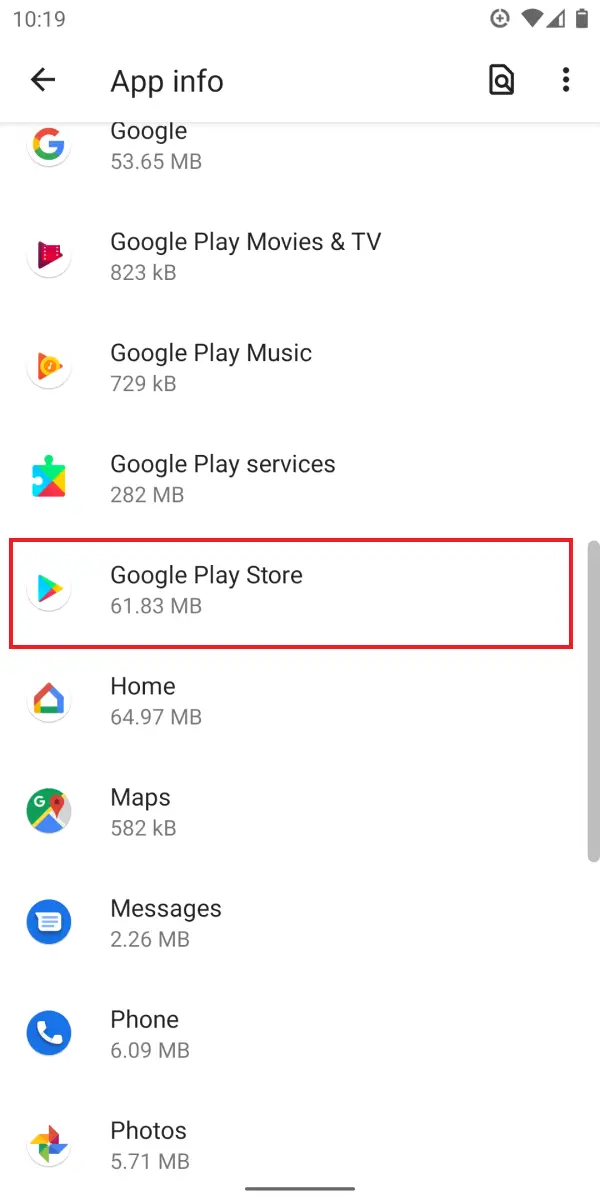Screenshot of a smartphone home screen captured at 10:19, displaying several system icons along the top status bar including Wi-Fi, data, and battery symbols. On the upper left, a back arrow and "App Info" are visible, beneath which an app page is presented with a search magnifier icon and three vertical black dots. The app list showing various applications is detailed as follows:

- Google: 53.65 MB
- Google Play Movies & TV: 823 KB
- Google Play Music: 729 KB
- Google Play Services: 282 MB
- Google Play Store: 61.83 MB (highlighted with a red box)
- Home: 64.97 MB
- Maps: 582 KB
- Messages: 2.26 MB
- Phone: 6.09 MB
- Photos: 5.71 MB

At the bottom, a black scroll bar offers navigation. On the left side, corresponding app icons are visible: a red Google triangle, a puzzle piece, a multicolored triangle, a multicolored envelope, the Google Maps symbol, a white text box in a blue circle, a white phone in a blue circle, and a multicolored pinwheel in a white circle. The interface appears to be in a settings or application management mode, with the focus on the "Google Play Store" app.